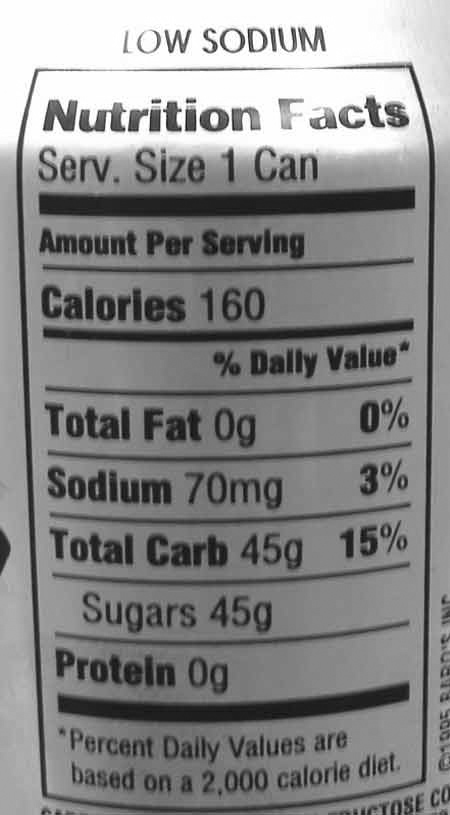The image is a close-up of a nutrition facts label on the back of a can, likely a beverage such as soda. The label consists of black text and lines on a white background. Just above the table, it is marked "low sodium." The table is slightly out of focus but clearly readable. The header reads "Nutrition Facts," followed by the serving size, which is listed as "1 can." The details under "Amount per serving" include: Calories - 160, Total Fat - 0 grams (0% DV), Sodium - 70 milligrams (3% DV), Total Carbohydrates - 45 grams (15% DV), all of which are sugars, and Protein - 0 grams. An asterisk notes that the percent daily values are based on a 2,000 calorie diet. There appears to be some additional, unreadable text cut off at the bottom of the label.